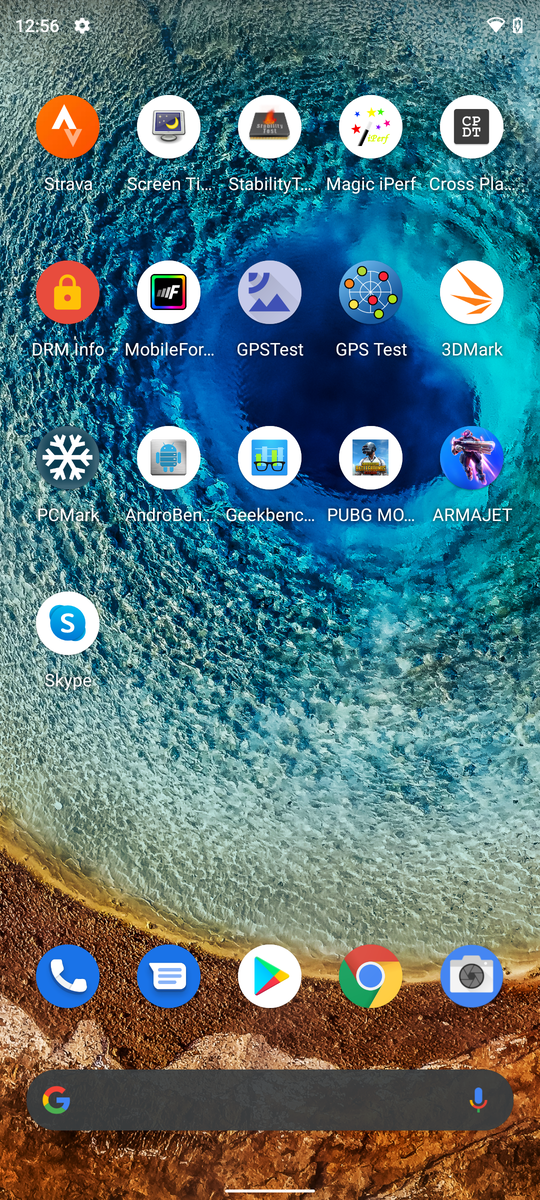A detailed screenshot of a smartphone home page displaying an intricate background, reminiscent of a blue geode or a sulfur pool. The centerpiece is a dark blue circle emitting radiant blue light, creating the illusion of a liquid surface with a hint of brown around the edges.

On the home page, we see a variety of apps arranged in a grid. These apps include Strava, a fitness tracking app; 'Screen' and 'Stability,' likely referring to system functions or tests; 'Magic I Perf,' and 'Cross Play,' both potentially related to performance benchmarking or gaming. Additionally, there are apps like DRM Info, GPS Test (appearing twice with different icons), 3DMark, PCMark, AndroBench, and GeekBench, which are all typically used for device testing or benchmarking. Other notable apps include PUBG Mobile, Armageddon, and Skype.

Below the grid of apps, the dock at the bottom of the screen features essential quick-access icons: a phone symbol for calls, an envelope symbol for emails or messaging, the Google Play Store, Google Chrome, and a camera icon which likely provides access to the phone's camera or gallery.